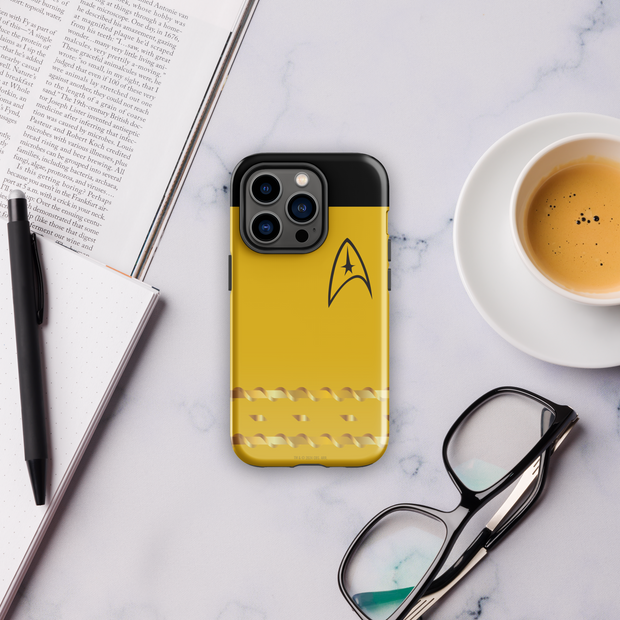This color photograph captures a top-down view of a white marble table cluttered with various objects. Dominating the center of the composition, a cell phone lies face down, showcasing its distinctive cover. The phone case is primarily yellow with a black top section and features a small, black, bent triangle-like logo reminiscent of a Star Trek insignia. Adjacent to the phone, a pair of black eyeglasses rests. To the right, a white saucer holds a matching white cup filled with a tan liquid that resembles either a creamy soup or a caramel macchiato. On the left side of the table, a notebook with an accompanying pencil lies next to an open magazine article. Overall, the scene is a snapshot of a casual, perhaps productive moment amidst everyday life.